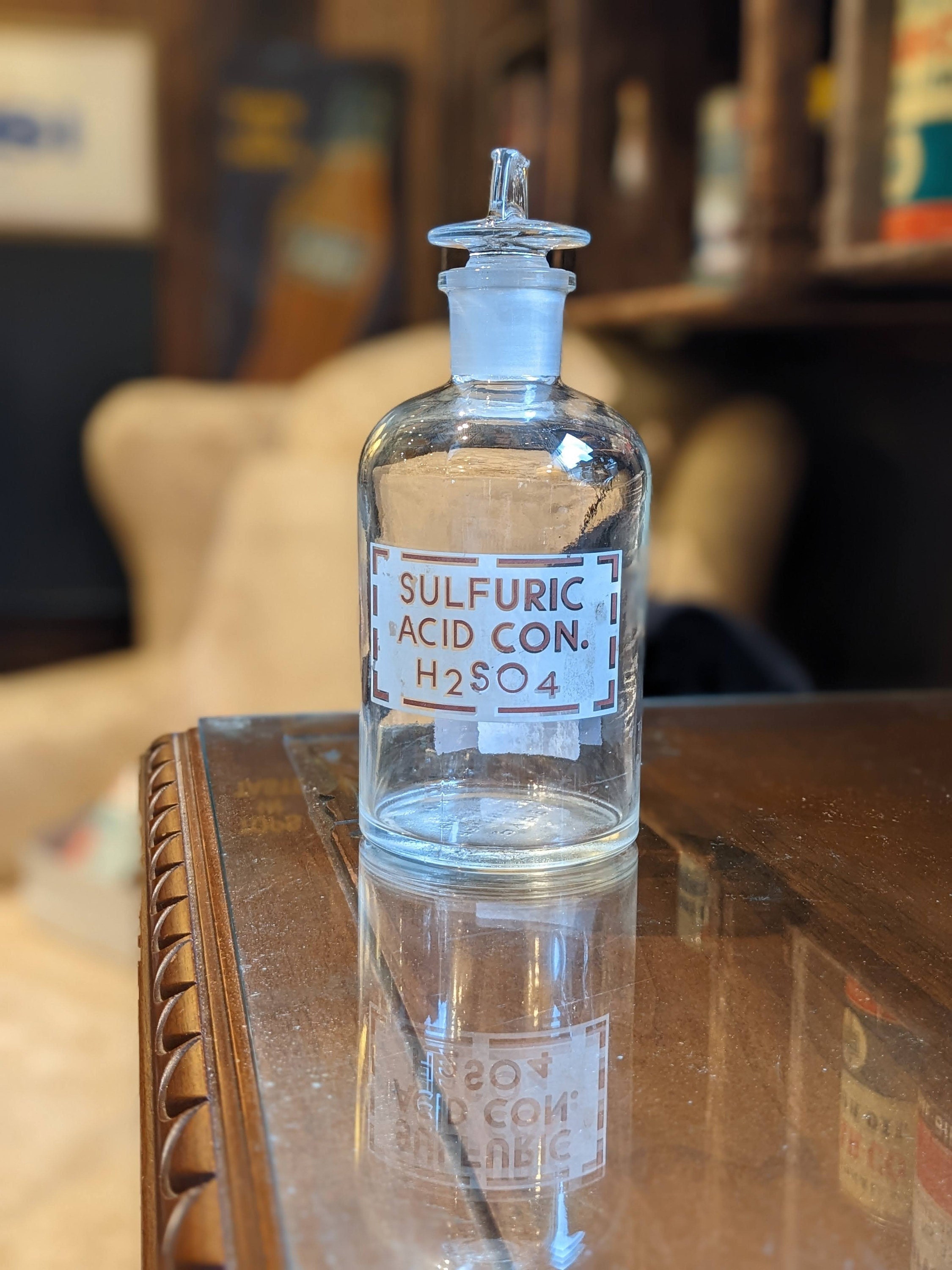This detailed close-up photo captures an antique, large glass bottle of sulfuric acid concentrate, meticulously designed with a frosted glass neck and a glass pull topper, complemented by a glass stopper with a rubber edge. The bottle, which is empty and in mint condition, features an etched label bearing the inscription "Sulfuric Acid Con H2SO4" on a striking white background. It is elegantly perched on a scalloped edge wooden desk with a glass top. The blurred background reveals a cozy study area adorned with a cream-colored winged chair, wood-paneled walls, and wood shelves lined with various indistinct items and posters leaning against the wall, enhancing the scene's antique and scholarly ambiance.